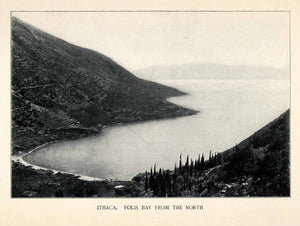This small, rectangular, black-and-white photograph, measuring approximately an inch and a half to two inches wide by an inch and a quarter high, features an off-white, eggshell-colored border that is thinner at the top and sides and slightly whiter at the base. The photograph depicts a bay, with water entering from the right-hand side and extending towards the lower left, rising up to the upper left-hand corner. The surrounding landscape includes mountains and hills covered with trees, alongside a small, white, sandy beach visible in the bottom left corner. The sky above appears to be clear or slightly cloudy, with a gray hue. At the base of the photograph, there is a black stamping that is difficult to read completely, but it seems to say "Poles Bay from the north."